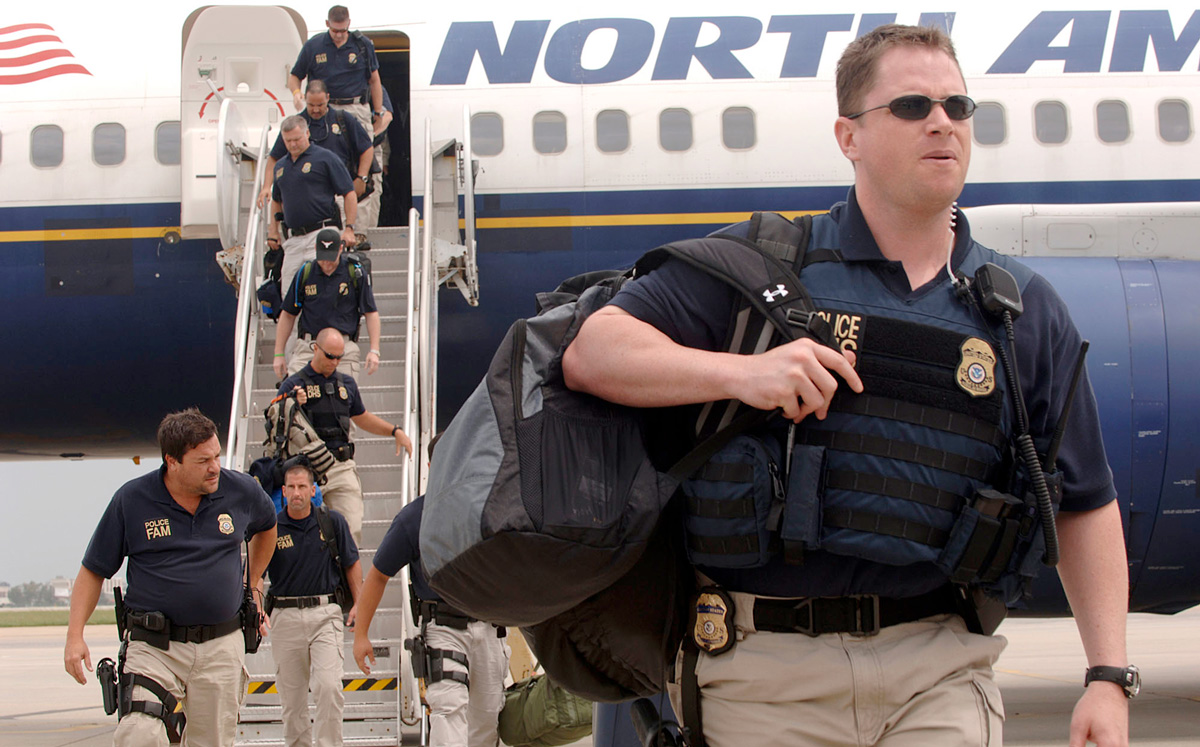In this detailed color photograph, multiple police officers are deplaning from a North American jet situated on a tarmac. The image is in landscape orientation, capturing officers in navy blue polo shirts with "Police Fam" partially visible on their attire, and traditional light tan khaki pants. The officers, mostly male, are descending aircraft steps with the closest individual to the viewer placed slightly right of center. This officer, with short brown hair and oval sunglasses, is depicted from head to mid-thigh, donning a dark collared shirt covered by a protective blue vest adorned with a badge on the left shoulder and embroidered "police" text partially visible on the right shoulder. He carries a black-strapped bag over his shoulder, with a gold badge affixed to a brown belt and khaki shorts. This officer, along with eight similarly dressed colleagues—some equipped with additional gear and holstered weapons—is making their way down the stairs onto the runway. The background features the jet, which is white on the upper half and blue on the lower half, marked with windows, a blue engine, and partially visible text indicating "North AM." The exterior environment appears gray and overcast, enhancing the detailed realism of the scene.